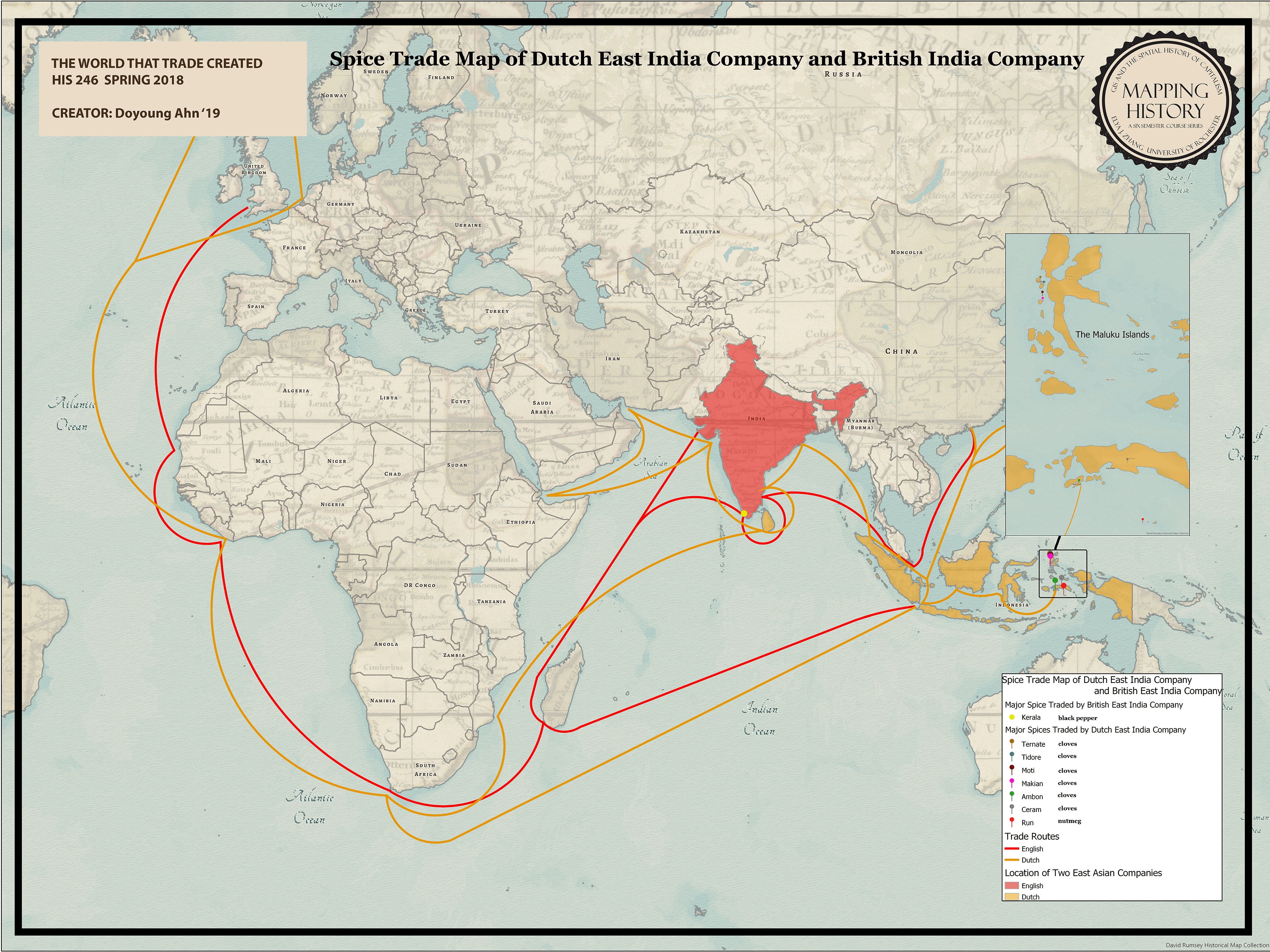This horizontal rectangular image is a detailed map of the spice trade routes established by the Dutch East India Company and the British India Company. At the top, the text reads "Spice Trade Map of Dutch East India Company and British India Company," along with "Mapping History. The World that Trade Created, History 246, Spring 2016." The map prominently features the routes in orange emanating from India, highlighted centrally in an orange hue, and extending to various countries. Notably, the routes circumnavigate Africa and reach into Europe, illustrating the wide-ranging impact of these trading companies. Additional text on the map identifies key areas such as Sri Lanka (Ceylon) and the Dutch East Indies. Countries in gold are also marked on the right side of the map. A legend is present at the bottom right corner, though its details are too small to read. The map is primarily colored in shades of lightish orange, gray, blue, black, and white, decently showcasing geographical and historical aspects of the spice trade.